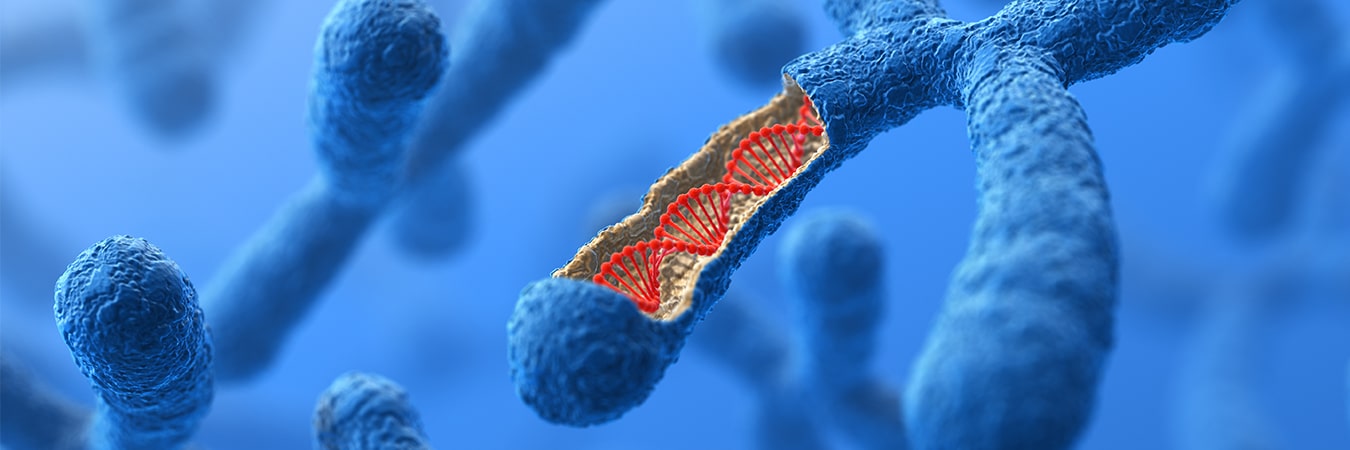This image appears to be a highly detailed and colored illustration of a microscopic view of cells or bacteria, specifically focusing on a chromosome. Set in a horizontal rectangle with a light blue background, the composition features multiple X-shaped chromosomes scattered throughout, with all but one being out of focus. The prominent X-shaped chromosome in the right-hand side is highlighted and appears in sharp focus. This chromosome extends beyond the top edge of the image with tubular sections reaching out in various directions.

Focusing on the detailed section, there is a midsection connecting two primary tubular appendages: one leading downward and to the left, and another falling almost straight down. In addition, there are appendages extending upwards and out of the frame. Notably, the downward and leftward extending section is illustrated with its top side removed, offering a view inside the chromosome. This reveals a red double-stranded DNA helix within a tannish membrane.

For an illustrative touch, the internal structure of the chromosome is portrayed as having red, fan-like DNA strands, potentially hinting at the intricate nature of genetic material. The visual content emphasizes the detailed, vibrant red double spiral of DNA against the beige-tinted cell wall, standing out dramatically within the chromosome cutout. The entire illustration suggests a blend of scientific visualization and artistic rendering, emphasizing the microscopic scale and complex structures of genetic material.